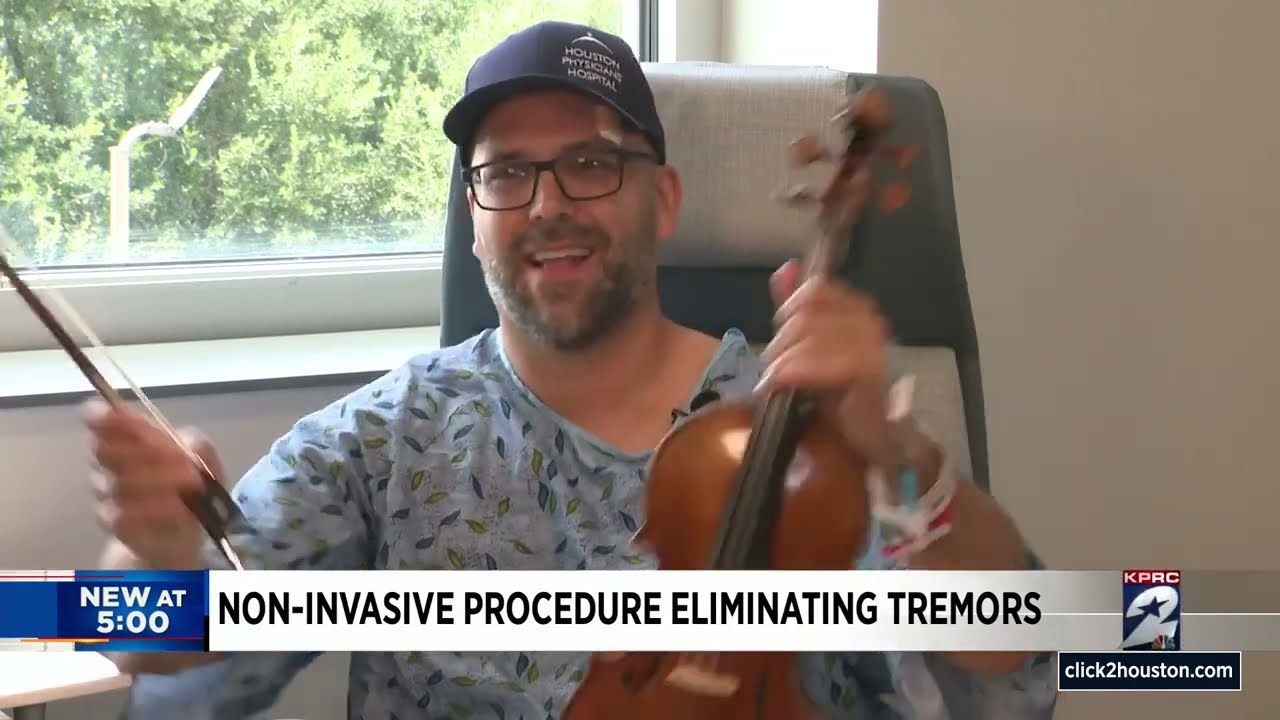The image is a still from a TV news broadcast about a public interest segment on KPRC 2, focusing on a non-invasive procedure for eliminating tremors. The screenshot prominently features a man in a hospital gown sitting in a gray and white chair, evidently in a medical setting. He sports a full beard, mustache, black-framed eyeglasses, and a blue baseball cap that reads “Houston Physicians Hospital.” He appears to be playing a violin or viola, holding the instrument in his left hand and the bow in his right. His mouth is open, suggesting he is speaking. Medical bands are visible on his left arm, indicating he might be undergoing treatment. Behind him, beige walls and a window through which a tree-filled landscape can be seen add context to the hospital environment. The text overlay on the image includes a blue box on the bottom left that reads "new at 5" and a white box with black text stating "non-invasive procedure eliminating tremors," followed by "KPRC 2" and "click2houston.com" in a black box below the channel number.